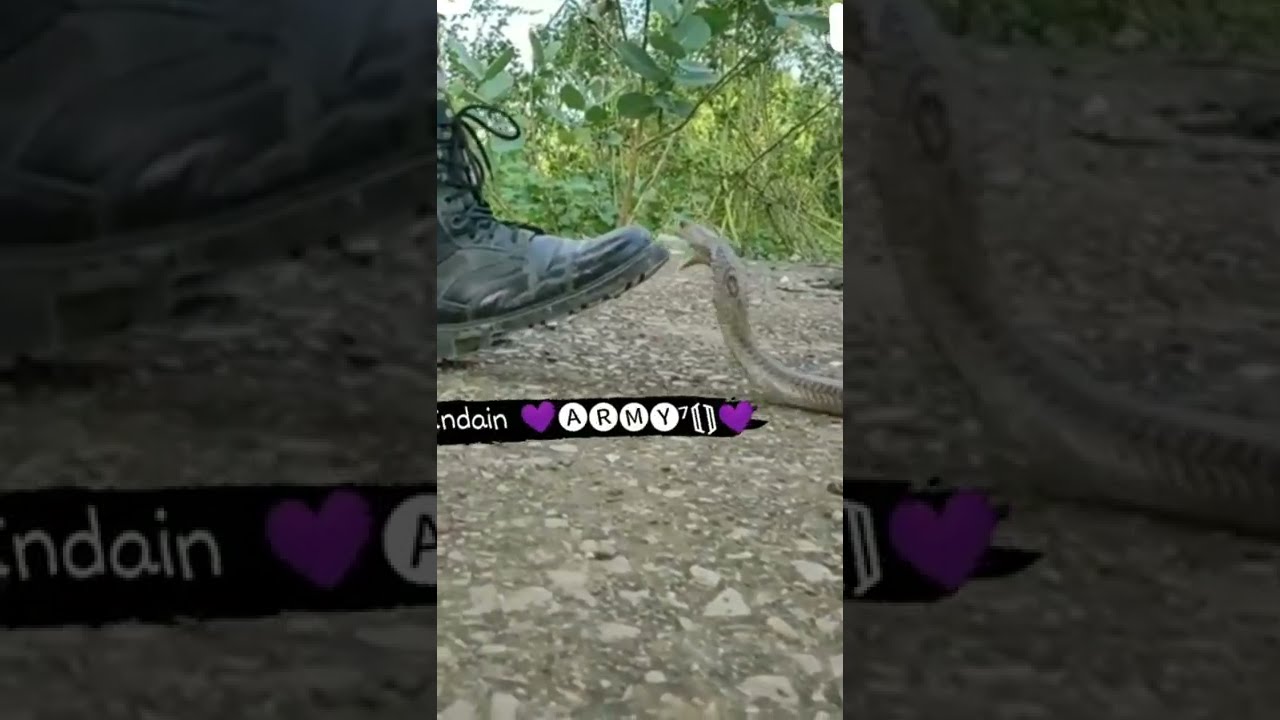The image is a color, outdoor photograph taken with a cell phone, capturing a striking moment between a snake and a boot. The boot, black with laces and resembling either a hiking or jungle boot, is positioned toe-up, held as if tempting a snake. The snake, possibly a cobra or rattlesnake, is grayish-brown and appears to be in mid-strike towards the boot, mouth open. The scene is set on a gravel footpath or road, with green vegetation visible in the background. Across the middle of the image is an illustrated black ribbon with white circular designs. The text on the ribbon is partially visible, showing "N-D-A-I-N" followed by a purple heart, the word "ARMY" in black letters within white circles, and then another purple heart. There are additional white symbols surrounding the "ARMY" text. The natural daylight enhances the vividness of the scene, highlighting the textures and colors of both the boot and the snake.